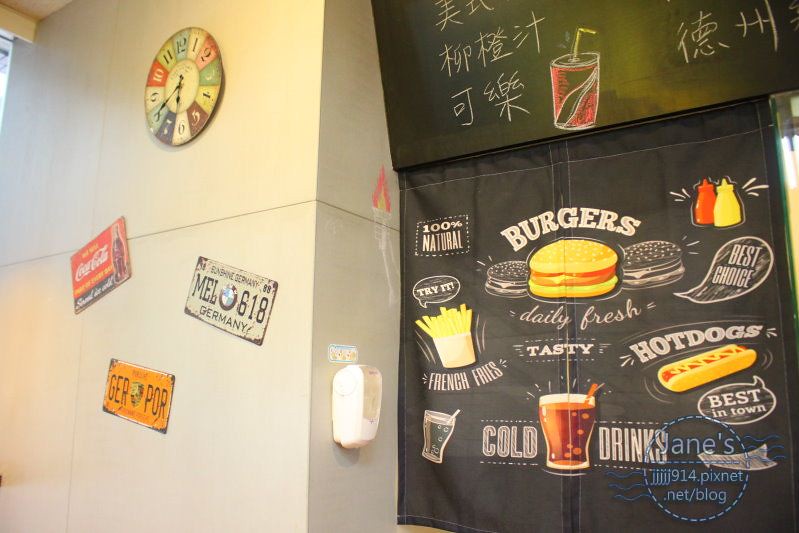This photograph appears to be taken inside a restaurant, capturing a richly detailed scene divided into two distinct sections. On the left side of the image, there is a colorful clock with its numbers one through twelve each in a different color, including shades of white, pink, green, yellow, brown, dark blue, light blue, red, gray, and blue. Below the clock, the white plaster wall is adorned with a hand sanitizer dispenser and several license plates, one from Germany marked “GER,” “MEL,” and "618" with a BMW symbol, and another plate featuring "P-O-R" with a shield-like symbol. An old tin Coca-Cola advertising sign with a distinctive Coca-Cola bottle is also mounted on this side of the wall.

On the right side of the photograph, there is a blackboard-like section with Chinese characters at the top and an intricate chalk drawing of a drink with a straw. Below this, there is a vivid illustrated banner or curtain with multiple food items and promotional text. The banner vividly displays images of burgers, hot dogs, french fries, and various condiments like ketchup and mustard. It includes enticing text such as “100% Natural Burgers,” “Daily Fresh,” “Tasty French Fries,” “Cold Drinks,” “Best in Town,” and “Best Choice.” These phrases appear in various fonts and colors, enhancing the lively and dynamic feel of the restaurant environment.